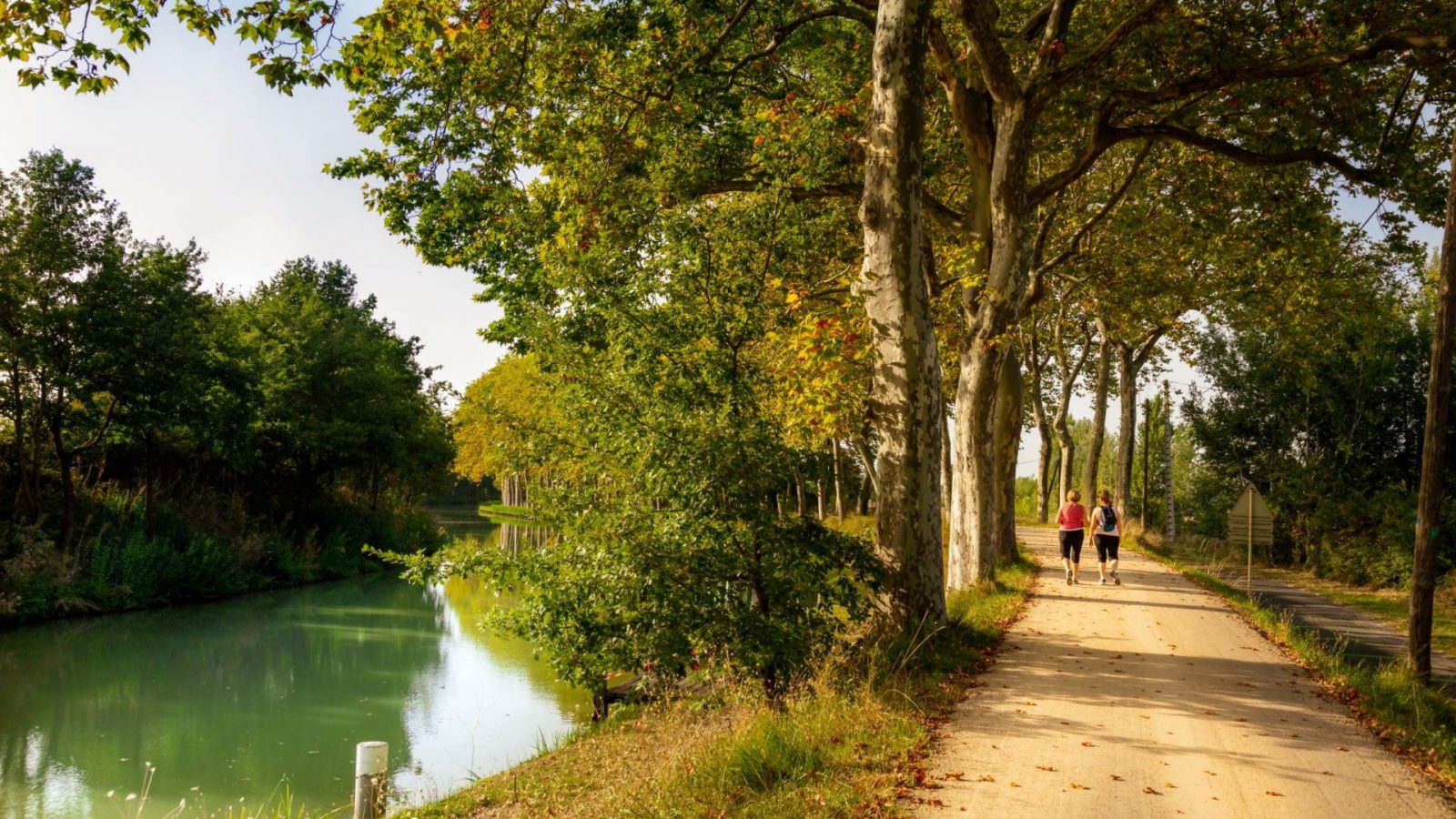The photograph captures a serene natural trail, endowed with the vividness of a sunlit day. The trail, possibly a paved path or even a wide dirt road with a light tan hue, stretches ahead, flanked by lush green foliage. Two women, donning capri-length leggings and t-shirts or tank tops, amble away from the viewer, one with a blue backpack. On the left, a tranquil body of water, perhaps a pond or a river with a greenish-brown tint, softly reflects the majestic green and yellowing trees, as well as the sun's rays. The water remains still, enhancing the peaceful ambiance. The right side of the trail is bordered by dense trees, possibly sycamores, their leaves a mix of rich green and some hints of yellow. This picturesque scene, likely set in a park, is a harmonious blend of nature's serene elements.